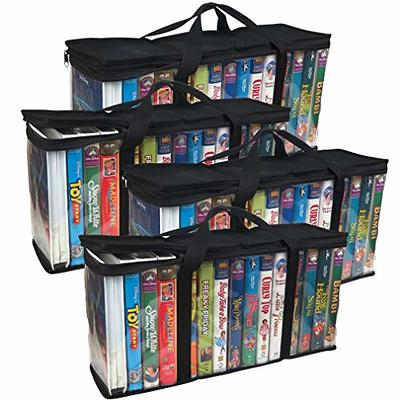The image depicts a collection of four clear-sided, rectangular cases designed to hold VHS tapes, each with black zippered tops and bottoms, and two sturdy canvas handles. The four cases are visually identical, suggesting the same image has been repeated or duplicated multiple times on a plain white background. Each case is filled with what appear to be popular Disney and children's movies, meticulously arranged in the same order. The visible titles include Toy Story, Snow White, Madeline, Freaky Friday, Mary Poppins, The Rescuers, Curly Sue, Fox and the Hound, and Bambi. Some of the VHS tapes are partially obscured by the canvas straps, making a few titles difficult to discern. The cases allow viewers to see the contents while offering a convenient way to carry the videotape collection. Two of the cases are shown open, while the other two are closed, adding variation to the repetitive arrangement.